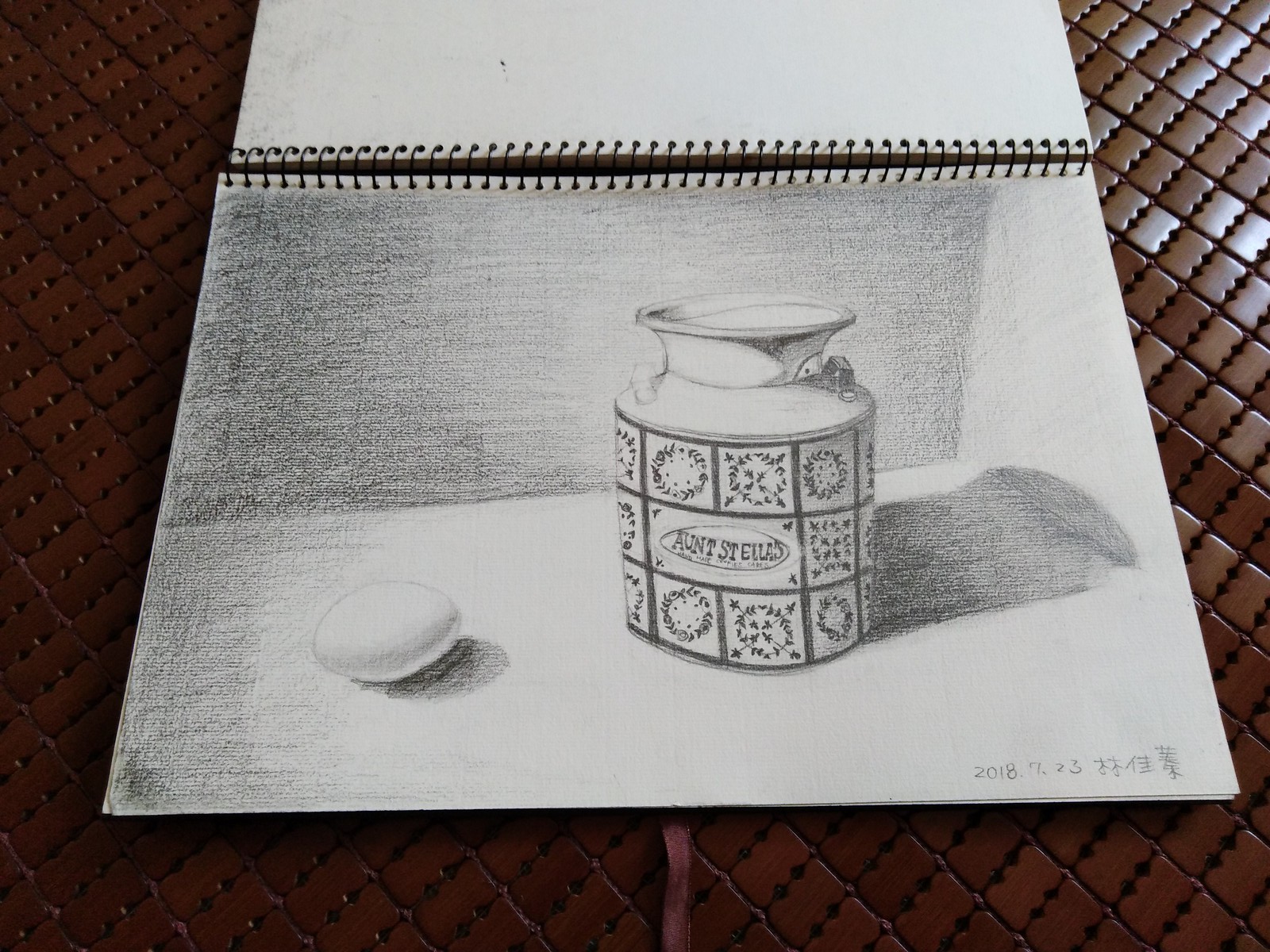The image showcases a white spiral-bound drawing pad resting on a brown, leather-like tabletop, characterized by a diamond-pattern cross-stitching and a reflective surface, particularly in the upper right-hand corner. The drawing pad, opened in landscape view, features a detailed pencil sketch of an old metal milk container positioned centrally. This container is adorned with decorative squares containing leaf wreaths and bears an oval label inscribed with "Aunt Stella's." To the left of the milk container, there is a carefully drawn egg. The sketch also includes the year "2018" and some additional text in a different language at the bottom. Overall, the foreground sketch appears to be rendered in either charcoal or pencil, capturing both the objects with intricate detail and shading.